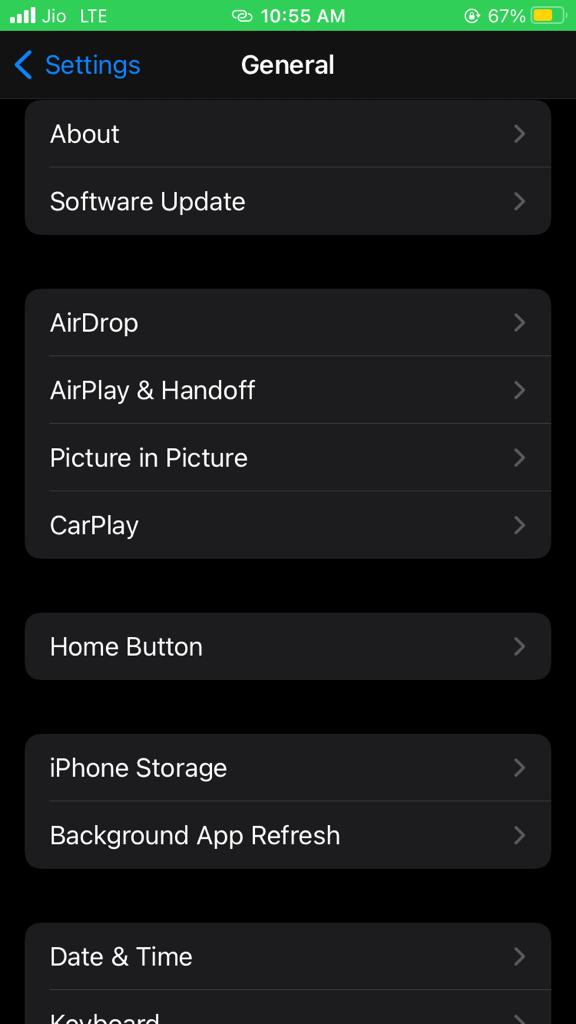The image showcases the screen of a device with a user interface containing various elements. At the top, there's a green status bar extending from left to right. On the left side of this bar, a cellular signal icon is visible, followed by the text "JIO," which is spelled J-I-O, and then "LTE." Positioned centrally in the green bar, the time is displayed as "10:55 AM." On the right side, there is a lock icon and the text "67%" indicating battery percentage, followed by a battery icon that contains a yellow bar representing the current battery level.

Just below the green bar, on the left side of the screen, there's a blue arrow pointing to the left, likely indicating a back button. On the right beside it, the screen displays the text "Settings," and further to the right, it reads "General."

Below this navigation section, a vertical list of tabs is presented, each representing different settings options. From top to bottom, the tabs are labeled as follows:
1. About
2. Software Update
3. AirDrop
4. AirPlay and Handoff
5. Picture-in-Picture
6. CarPlay
7. Home Button

This detailed configuration screen suggests that the image was taken while the user was navigating through the general settings of their device.